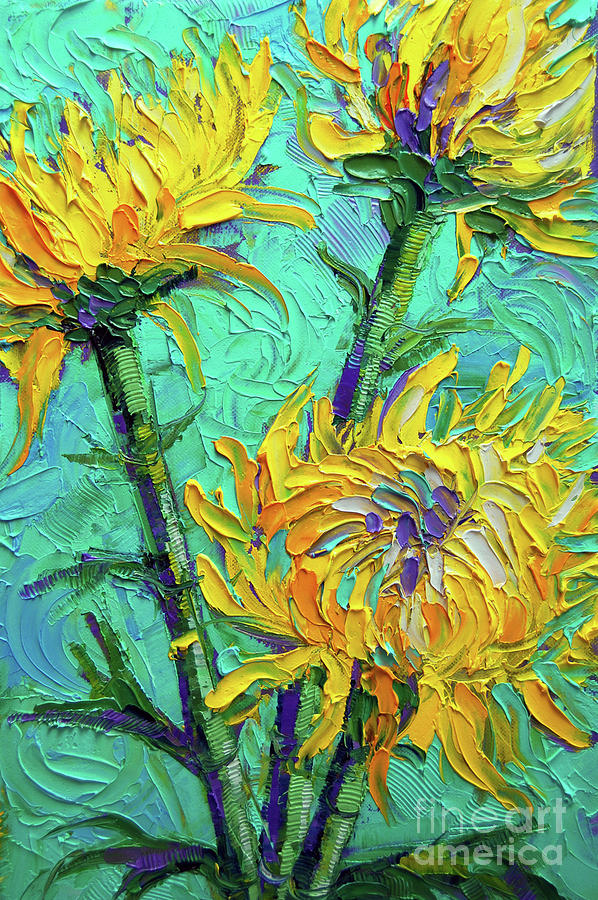The painting features a vibrant and textured depiction of three yellow flowers with bushy, mum-like petals, rendered with thick, expressive brush strokes. The petals exhibit a range of colors from yellows to oranges, with accents of white. The flower centers reveal hints of blue and purple, adding depth to the composition. The flowers extend from long green stems that occasionally show branches with shades of purple and various greens. The background is a light turquoise, reminiscent of a clear sky, with noticeable brush strokes that enhance the painting's tactile quality. The stems display lines that seem to have been scratched into the paint, offering an additional layer of texture. One flower on the right is shorter, another in the center reaches the top right corner, and the third on the left almost touches the top left corner. In white lettering, the bottom right corner reads "Fine Art America," marking the piece's artistic origin.